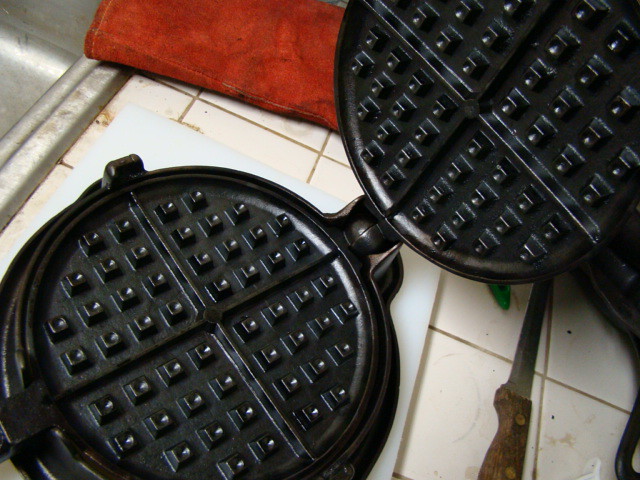The image captures a close-up view of a dirty white-tiled kitchen counter. In the center, there is a prominent black waffle maker, which is open, revealing four quadrants where the waffle pieces would form. The black cast iron surface of the waffle maker contrasts with the grimy white tiles that have brown, dirty grout. On the right side of the image, a sharp knife with a wooden handle lies near the edge of the counter. In the background, above the waffle maker, there is a red item that appears to be either an oven mitt or a towel. Partially visible in the top left corner is what seems to be the edge of a silver sink, indicating that this scene is taking place in a kitchen.